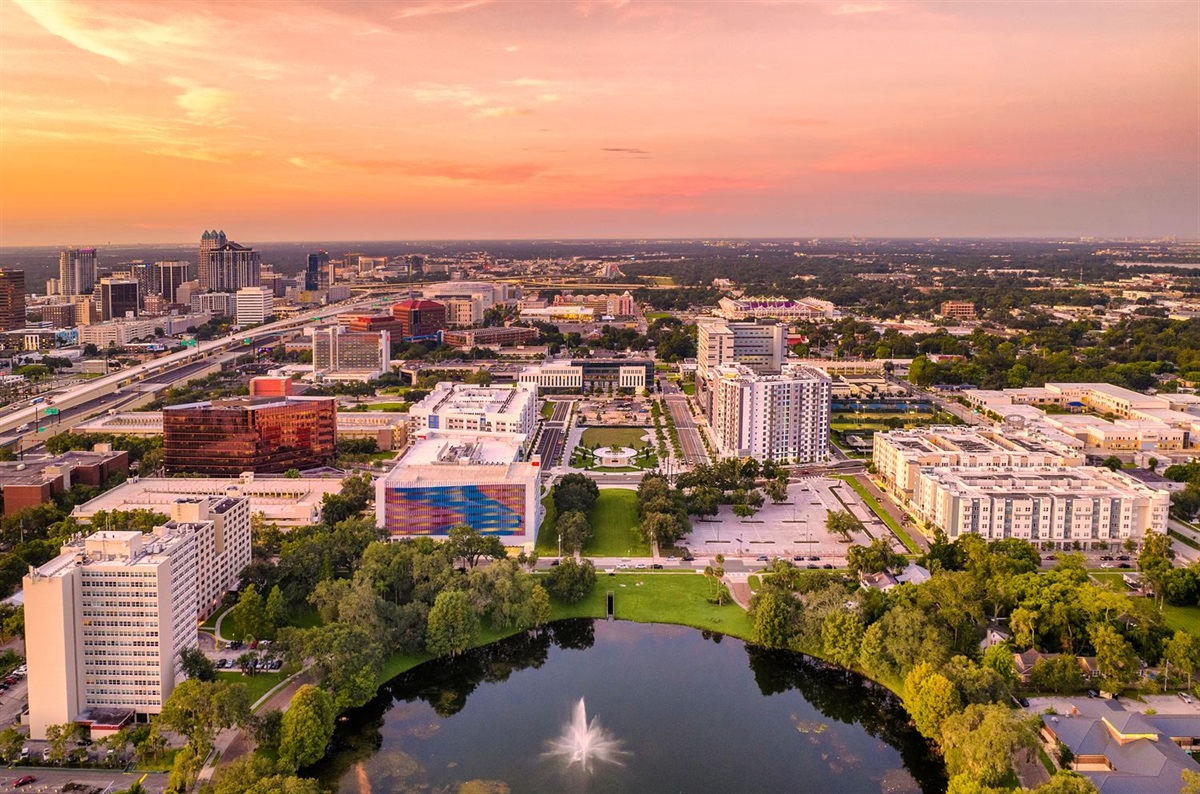This is an aerial view of a small city at either sunrise or sunset, characterized by a striking horizon line that transitions from light gray to stunning shades of amber, purple, orange, yellow, peach, and salmon. The image prominently features a large, human-made pond situated at the very bottom center, nestled within a lush park framed by verdant green grass and clusters of trees. At the heart of the pond, there's a fountain with a white spray rising into the air.

To the left of the pond stands a substantial multi-story office or apartment building, with various other white buildings scattered throughout individual blocks as the cityscape extends into the distance. Notable among the white and tan architecture is one building adorned with salmon-colored graffiti accented with blue, and another building entirely in red, with a second small red building visible in the distant background.

The left side of the image also features a freeway, suggesting connectivity and movement within this sprawling urban area, which includes both downtown buildings and expanding suburbs. A parking lot can be seen across the street from the green patch surrounding the pond, enhancing the accessibility of this serene park area amidst the urban environment.